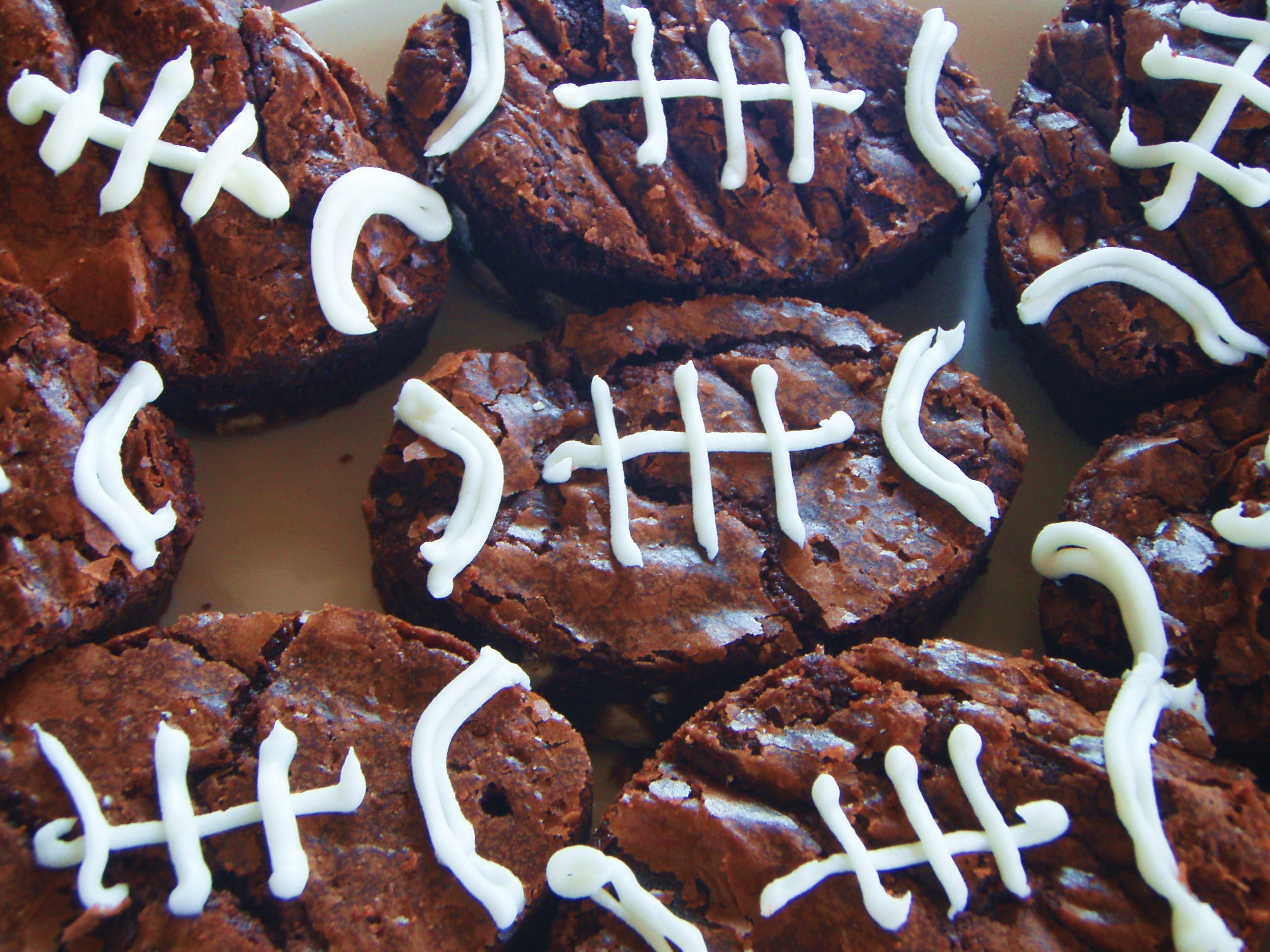The image is a photograph featuring a partially visible white plate adorned with several brown, oval-shaped desserts that resemble American footballs. The desserts, which appear to be thick brownies based on their smooth, caramelized surfaces, are meticulously decorated with white icing to mimic the stitching of footballs. The icing forms patterns that include a central horizontal line and three vertical lines intersecting it, giving the treats a distinctive look. The foreground displays one prominently placed dessert surrounded by seven others, also marked with similar stitching patterns. Notably, the brownies exhibit a slightly cracked surface, adding texture and authenticity to their appearance.